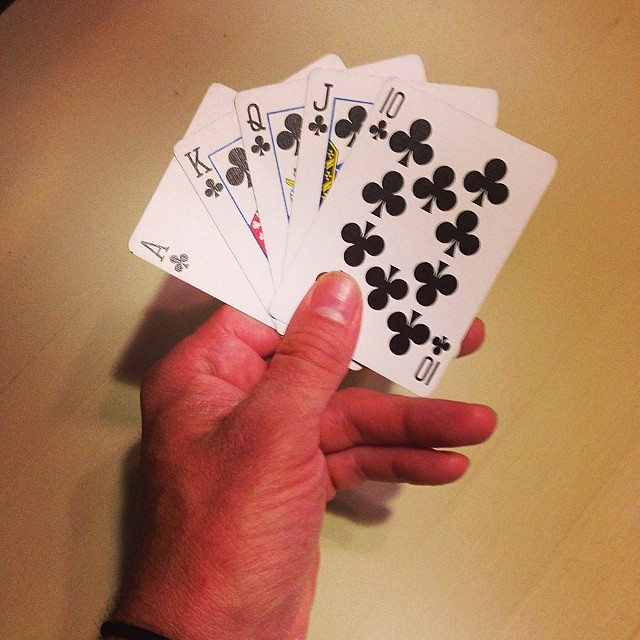The image showcases a close-up color photograph of a left hand holding a fan of playing cards. The background is blurred, presenting a brownish-gold hue that beautifully contrasts with the sharp focus of the cards and hand. The skin tone of the hand appears to be Caucasian, with the thumb prominently displayed, and the fingers are curled behind the cards, enhancing the grip. The cards are arranged in a fan-like spread from left to right, revealing five distinct Club cards. From the far left, the Ace of Clubs is followed by the King, then the Queen in the center, with the Jack next, and finally, the Ten of Clubs on the far right. The Ten of Clubs is the most visible, displaying nearly its entire face, save for the lower club symbol, which is partially obscured by the thumb. The cards are pristine and show no signs of wear, indicating they are new. There is a gentle shadow cast onto the background by the hand and cards, and a slight glare on the Ace of Clubs due to light reflection. This plays up the freshness and cleanliness of the playing cards, adding a touch of realism and texture to the photograph.